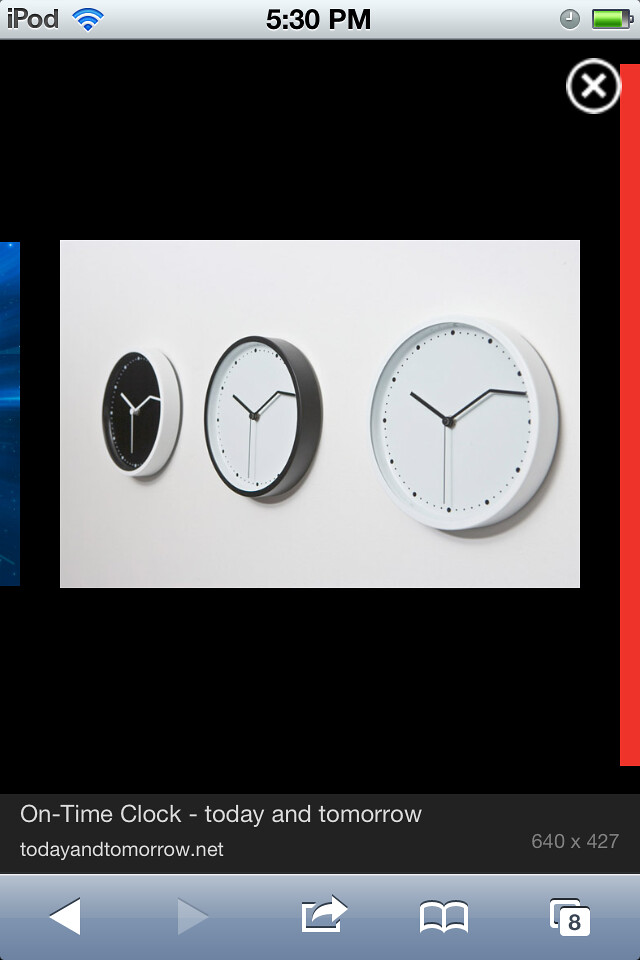The image appears to be a screenshot taken from an iPod. This is indicated by the "iPod" label at the top left corner, along with the Wi-Fi signal icon consisting of blue curves. The time displayed in the center is 5:30 PM, and the top right corner shows an almost full battery icon.

The main content of the screenshot features an image with a black background and a white rectangular frame in landscape orientation. The title of the image is "On Time Clock, Today and Tomorrow," and it is attributed to the website todayandtomorrow.net. The image size is specified as 640 by 427 pixels.

Within the white rectangle, there are three analog clocks, all showing approximately the same time, around 10:10 or 10:11, a common time used in advertisements. The clock on the far left has a black face with white hands and no numbers. The middle clock features a white face with black hands and a black rim around its edge. The clock on the far right has a white face with a white rim and black hands.